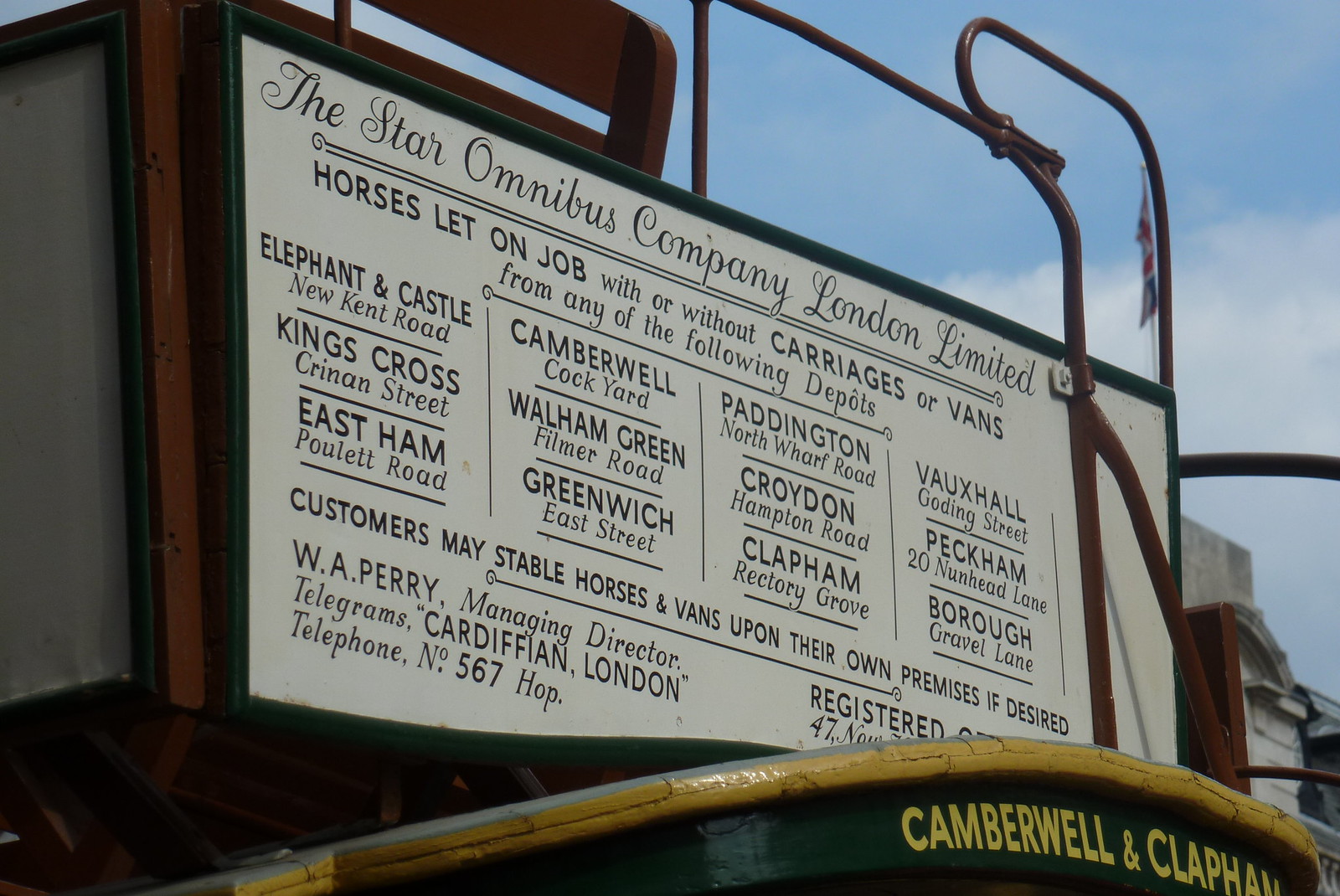The image showcases a large outdoor sign or banner, possibly mounted on a building or a vehicle, with a white background and bold black text. The sign advertises the Star Omnibus Company London Limited, managed by W. A. Perry, and provides details about their transportation services. It prominently states: "Horses let on job with or without carriages or vans from any of the following depots," followed by a comprehensive list of depots including Elephant and Castle, New Kent Road, King's Cross, Greenwich Street, East Ham, Poulet Road, Camberwell (Cock Yard), Wallum Green, Filmer Road, East Street, Paddington (North Wharf Road), Croydon (Hampton Road), Clapham (Rectory Grove), Bow Hall, Coding Street, Peckham (29 Nunhead Lane), and Borough (Gravel Lane). The sign also mentions that customers may stable horses and vans on their premises if desired. In the lower section, it provides contact information, including telegrams directed to Cardiff in London and a telephone number, 567.